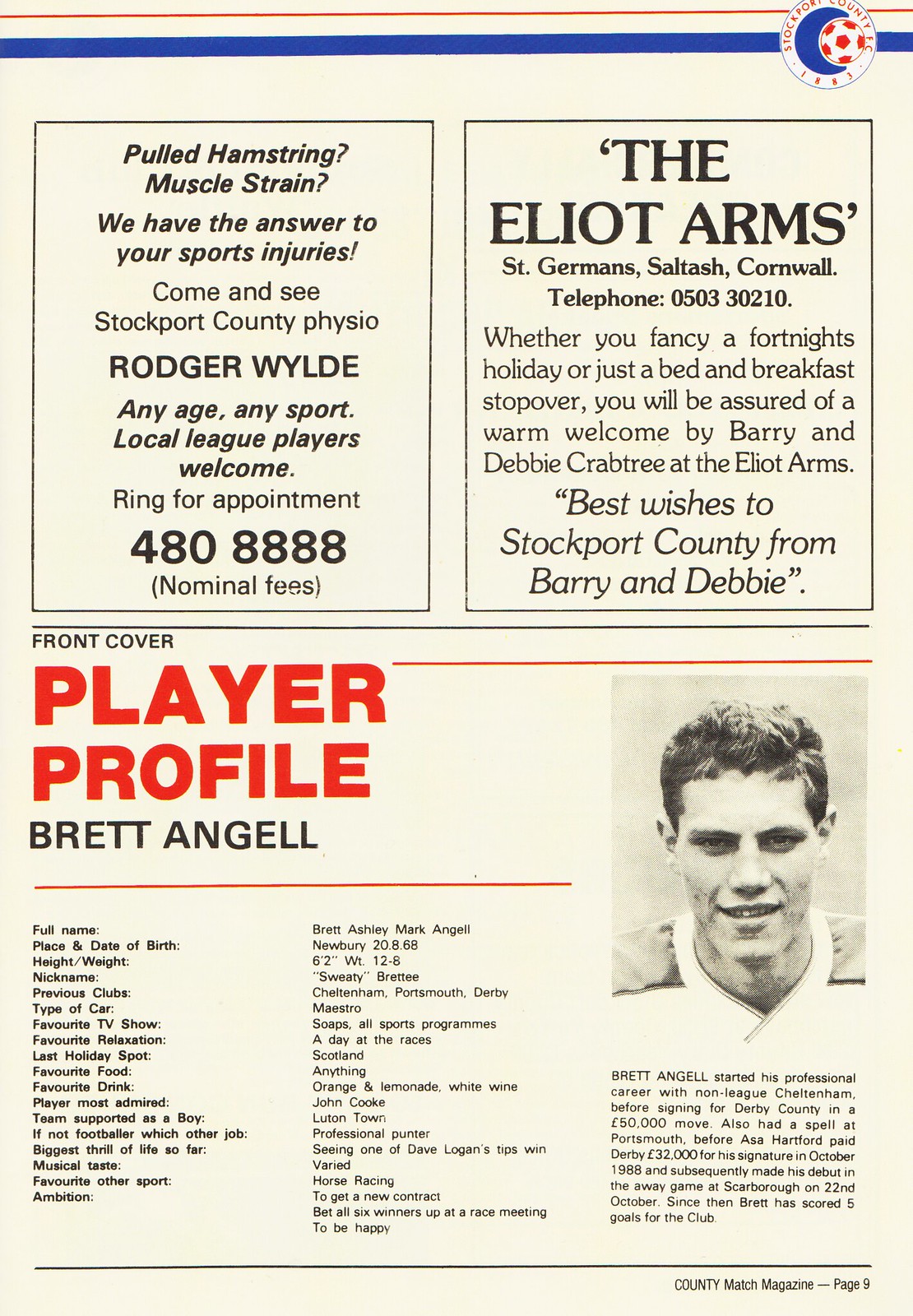The image showcases a page from County Match magazine, predominantly featuring an advertisement section and a player profile. The background exhibits a creamish hue with subtle greenish undertones. At the top of the page, there is a narrow blue band, topped by an even thinner red bar. In the upper right corner, there's a logo for Stockport County FC, which includes a red and white soccer ball and accompanying text.

The upper half of the image is divided into two rectangular text boxes. The left box contains an advertisement for Roger Wilde, addressing sports injuries with the message: "Pulled hamstring, muscle strain. We have the answer to your sports injuries. Come and see Stockport County Physio Roger Wilde. Any age, any sport, local league players welcome. Ring for an appointment at 480-8888. Nominal fees." The adjacent box on the right advertises The Elliott Arms, located in St. Germain's, Saltash, Cornwall. It reads: "Whether you fancy a fortnight's holiday or just a bed and breakfast stopover, you'll be assured of a warm welcome by Barry and Debbie Crabtree at The Elliott Arms. Best wishes to Stockport County from Barry and Debbie. Telephone: 0503-30210."

Beneath these advertisements is a thin black line labeled "front cover," followed by a prominent red text "Player Profile," and below it, in black, "Brett Engel." To the right, a grainy black-and-white photograph of Brett Engel accompanies the player profile, detailing his full name, place and date of birth, and additional personal information. This page appears on page nine of the magazine.